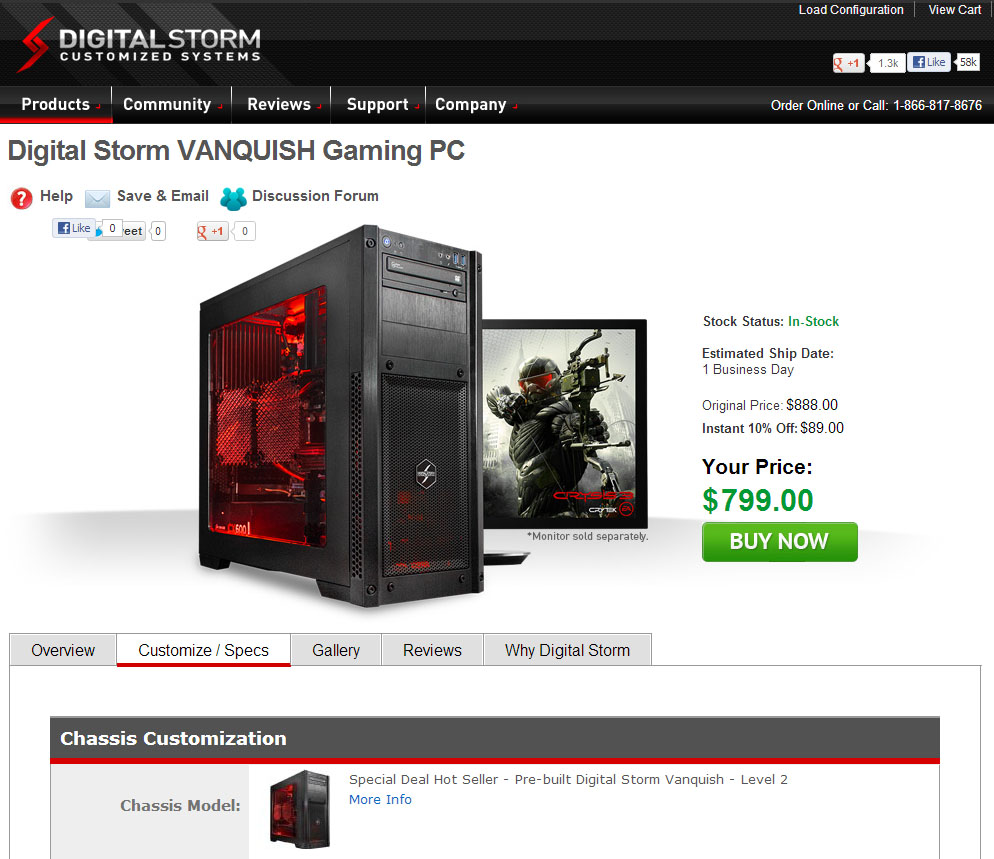Digital Storm Vanquish Gaming PC Product Page

This webpage highlights a high-performance gaming PC from Digital Storm, specifically the Vanquish model. The top of the page features a navigation bar with several tabs, including "Products," "Community," "Review," "Support," and "Company." Additionally, there are options to "Order Online" or call a phone number displayed near the top.

Prominent on the page is a large, striking image of the Digital Storm Vanquish Gaming PC. Immediately surrounding this image are various social media buttons linked to Google and Facebook, showcasing the number of likes they have received.

Key purchase information is prominently displayed: the gaming PC is currently in stock, with an estimated shipping date of one business day. The original price of $888 has an instant 10% discount applied, reducing the price to $799. A green "Buy Now" button is located below this pricing information.

Further down, there are several tabs to explore additional details about the product, including "Overview," "Customize/Specs," "Gallery," "Reviews,” and "Why Digital Storm." The "Customize/Specs" tab is active, revealing detailed information on the system's Chassis customization options. Specifically, it mentions the Chassis model as the "Special Dead Hot Seller," a pre-built Digital Storm Vanquish Level Two. 

Additionally, there's an option to click for more information, supplemented by another image of the gaming PC. The page also includes a handy "View Cart" option situated in the top right-hand corner for easy access to the shopping cart. 

This complete and immersive product page design ensures potential buyers have all the information they need to make an informed purchase.